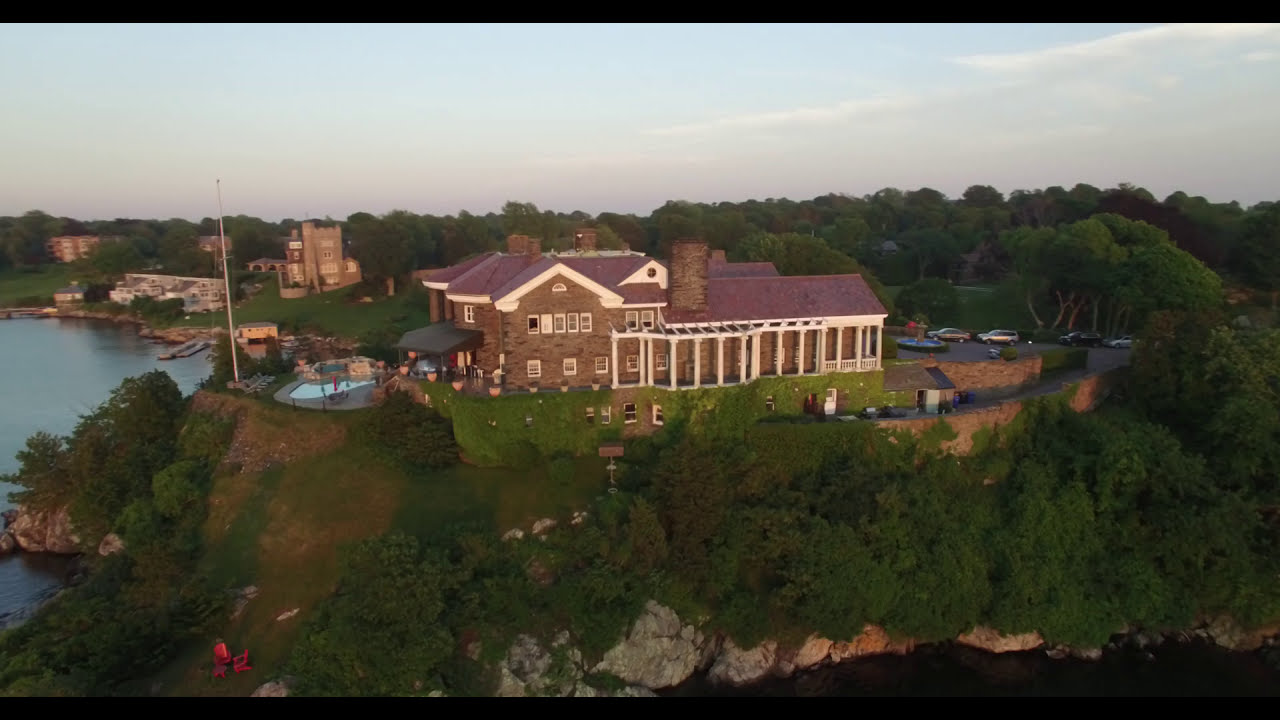The image depicts a grand, multi-story brick house built atop a rocky peninsula that juts out into a lake. The house, which could also be described as a large lodge, features a distinct red brick roof and is encircled by impressive white pillars, at least around its front half. The structure appears robust with large brick fireplaces and several chimneys, counted to be around four or five. It boasts luxurious amenities, including a massive in-ground pool with blue water and a gray cement deck, alongside a dark green or black awning. 

A striking brick wall forms the foundation on which the house is built. Surrounding the house, the landscape is lush with green trees and a beautifully manicured lawn that slopes gently down to the edge of the lake, presenting a picturesque descent though it might present some difficulty in the climb back up. Two red chairs and a small red table are placed near the foot of the hill, adding a touch of color to the green expanse.

The front of the house showcases a circular driveway or parking lot, adorned with a central fountain that has blue water, and is bordered by a black street top. Several high-end cars, including cream-colored, white, black, and silver vehicles, are parked here, suggesting a wealthy residential area. 

Adjacent to the house and visible in the background are other upscale homes, primarily tan or white with gray rooftops, enhancing the affluent neighborhood's aesthetic. The sky above is a serene blue with patches of white, while the heavily wooded backdrop further envelops the scene in natural beauty.